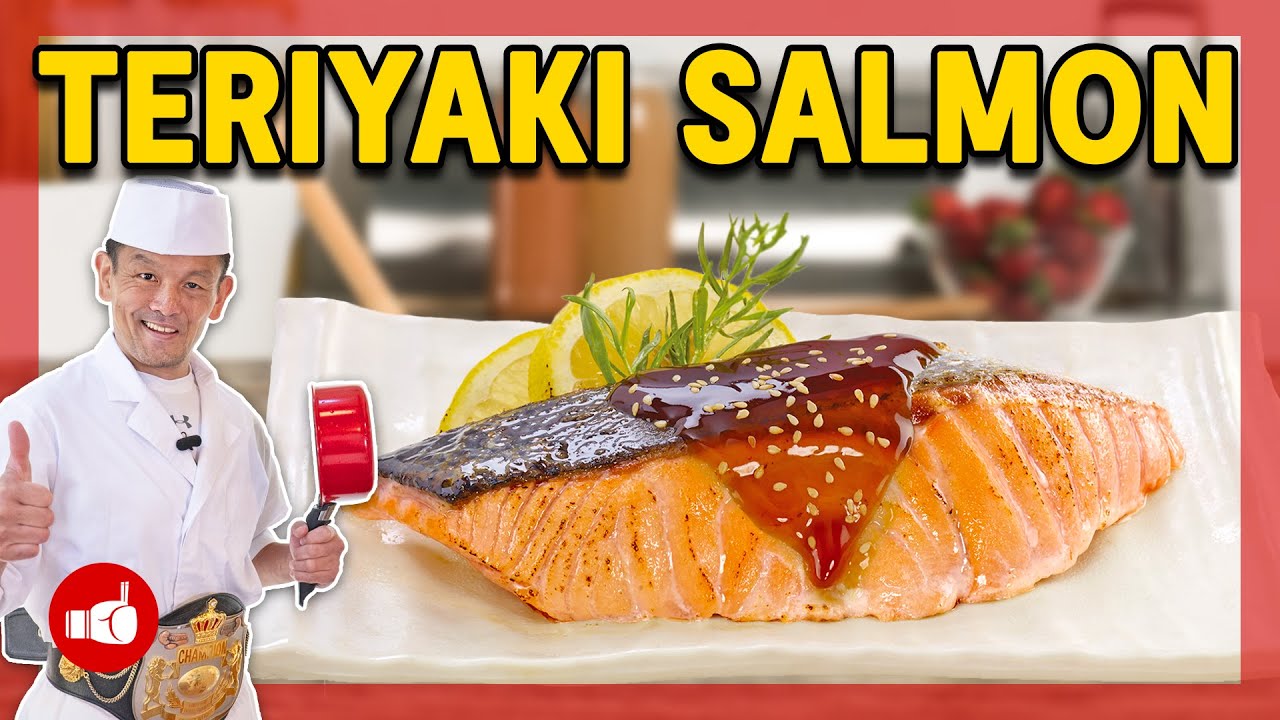This promotional photograph, potentially a YouTube thumbnail, features a well-cooked piece of Teriyaki Salmon garnished with sesame seeds and a rich glaze, prominently displayed on a flat, rectangular white plate. The plate includes two vibrant yellow lemon slices and a sprig of greenery, likely rosemary, positioned behind the salmon. The top of the image showcases bold, bright yellow text that reads "Teriyaki Salmon." On the left side, an Asian-looking gentleman, presumably the chef, stands smiling. He wears a white chef's coat, a flattened white hat, and a large ornate championship belt around his waist. His right hand gives a thumbs-up while his left holds a red saucepan. A small red circle logo depicting a white boxing glove holding chopsticks is located at the bottom left, adding a unique touch to the composition.